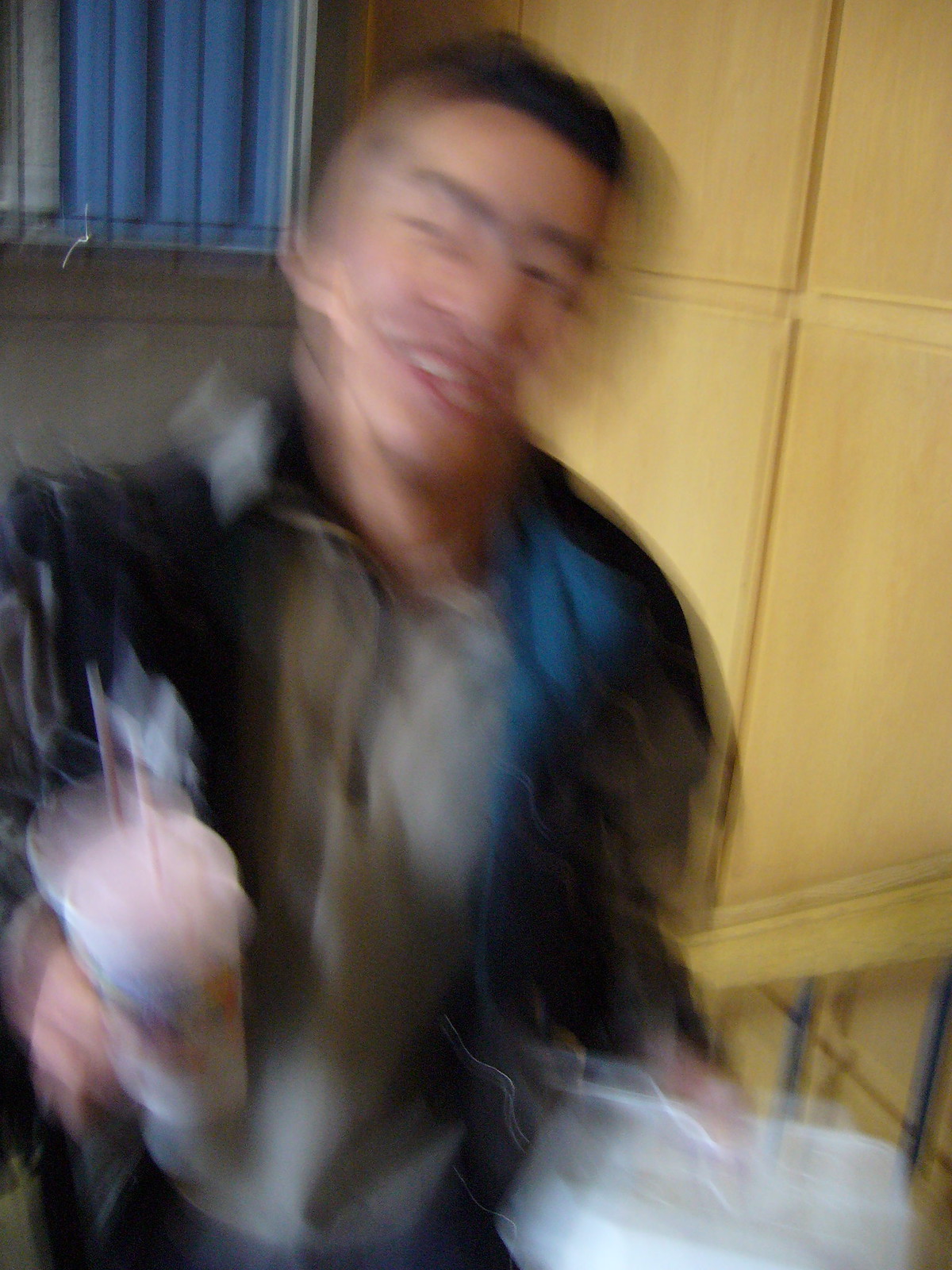In this blurred image, a dark-skinned gentleman is captured mid-smile, exuding happiness. Despite the lack of clarity causing some distortion, it's evident he's standing while holding a meal. In his right hand, he grasps a drink with a straw, and in his left, a white takeout container filled with food. He sports a stylish haircut, faded around the sides with dark hair on top. His attire includes a long-sleeve jacket layered over a collared shirt. The background showcases a tannish wood-colored wall, adding a warm tone to the scene.